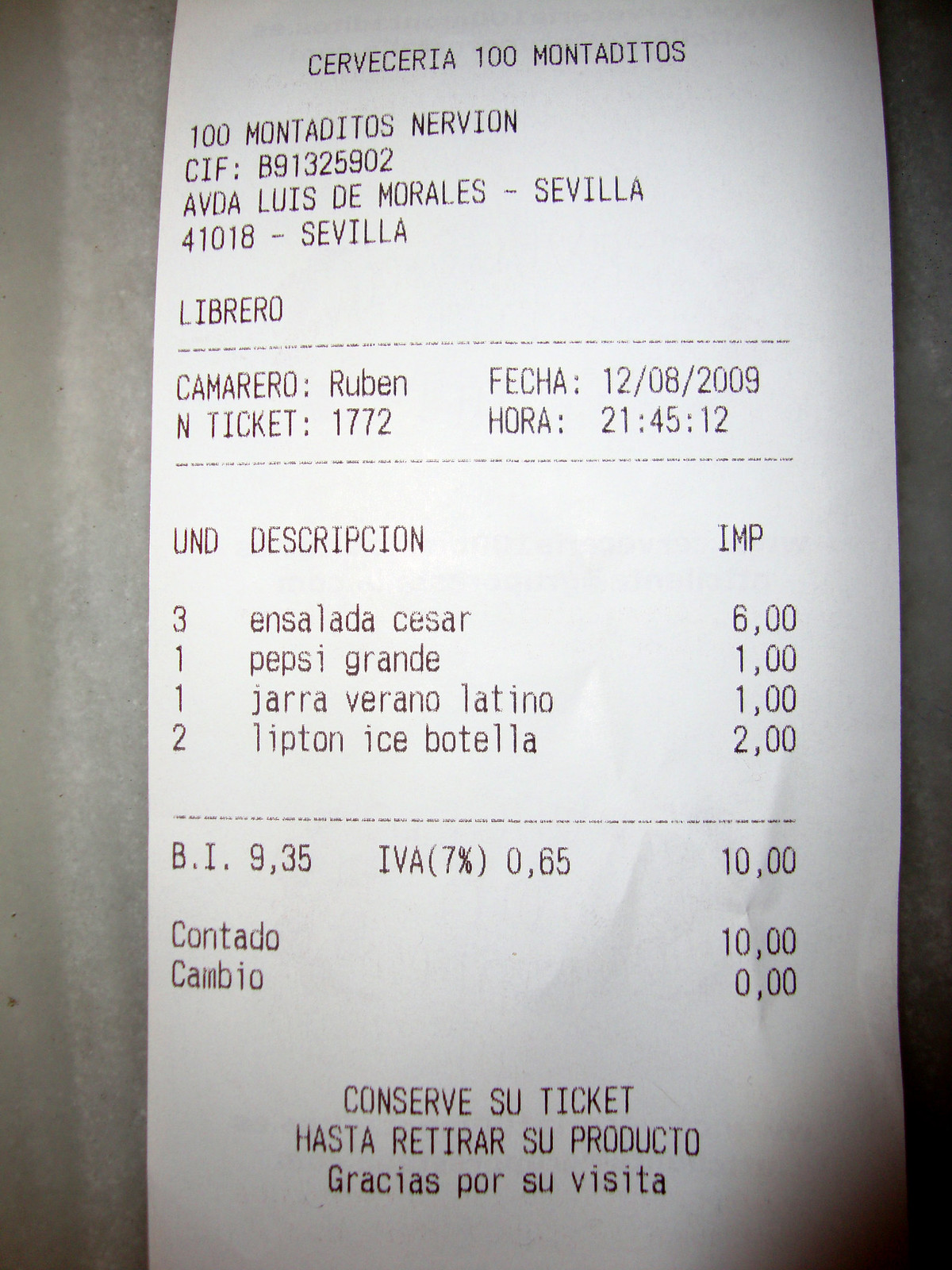This image depicts a detailed receipt from the restaurant "Cerveceria 100 Montaditos Nervion," located on Avda Luis de Morales, Sevilla. The cashier's name is Ruben, and the transaction occurred on December 8, 2009, at 21:45:12, under ticket number 1772. The items listed are three Caesar salads ("Ensalada Caesar"), one large Pepsi ("Pepsi Grande"), a pitcher of Verano Latino ("Jara Verano Latino"), and two bottles of Lipton iced tea ("Lipton Ice Botella"). The total amount for the order came to exactly 10, though the currency is not specified.